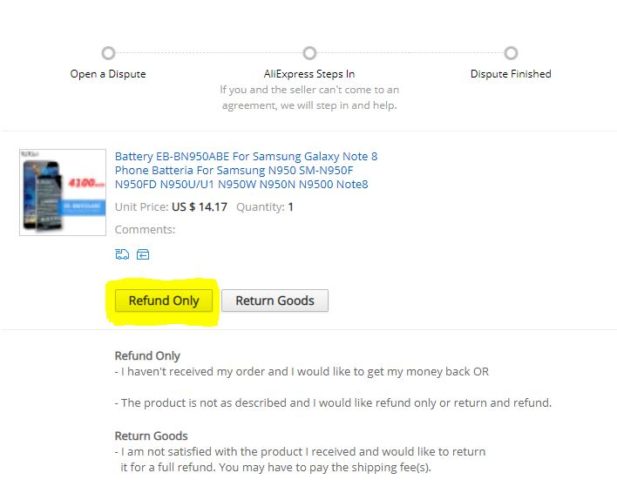In the image, the interface of an AliExpress dispute resolution process is shown. At the top, there's a circle labeled "Open a Dispute." Below that, a line connects to another circle stating, "AliExpress steps in: If you and the seller can't come to an agreement, we will step in and help." This is followed by another line ending in a circle labeled "Dispute Finished."

On the left side of the interface, there's a blurry image depicting the disputed item, which is not clearly visible. Next to it, detailed text reads: "Battery EB-BN950ABE for Samsung Galaxy Note 8. Phone battery for Samsung N950, SM-N950F, N950FD, N950U/U1, N950W, N950N, N9500, Note 8." The item's unit price is listed as $14.17 with a quantity of one.

Below this, there are two buttons for dispute resolution: "Refund Only" and "Return Goods." The "Refund Only" button is highlighted with a yellow marker effect, likely added through photo editing software, while the "Return Goods" button is displayed in gray with black font.